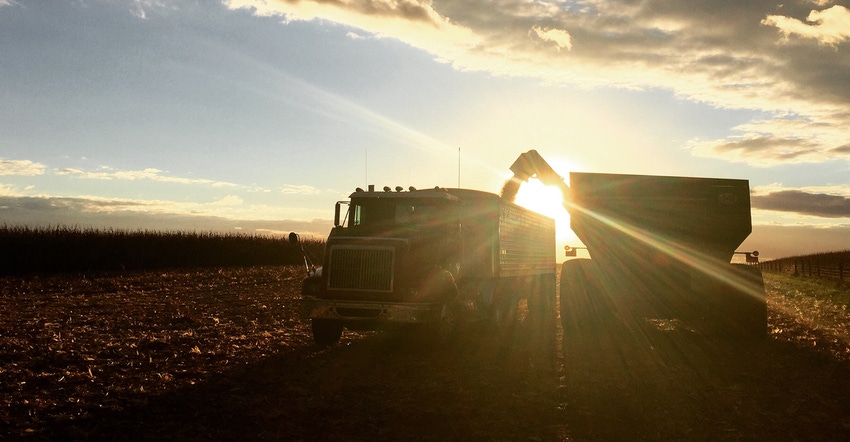The photograph captures a farming scene under a clear, beautiful blue sky with some clouds scattered mostly on the right side, extending slightly past the center. Below the sky, the image shows a recently harvested, open field. Positioned towards the right side of the field are two large farming vehicles. One of these is identified as a red semi-truck facing the camera, though it's partly obscured by shadows, making it difficult to discern details. Attached to this semi-truck is an extended trailer with an open top, presumably to catch grain or seed. Adjacent to this truck is another piece of farming machinery with an arm or feeder projecting from it, directing grain or seed into the trailer. The sun is setting behind these vehicles, casting light directly under the feeder arm, which enhances the dramatic effect but makes details of the arm somewhat indistinct. To the far left, beyond the barren field, there appear to be trees or another type of vegetation. On the right side of the image, some grass and what looks like a fence are visible, adding to the overall pastoral setting.